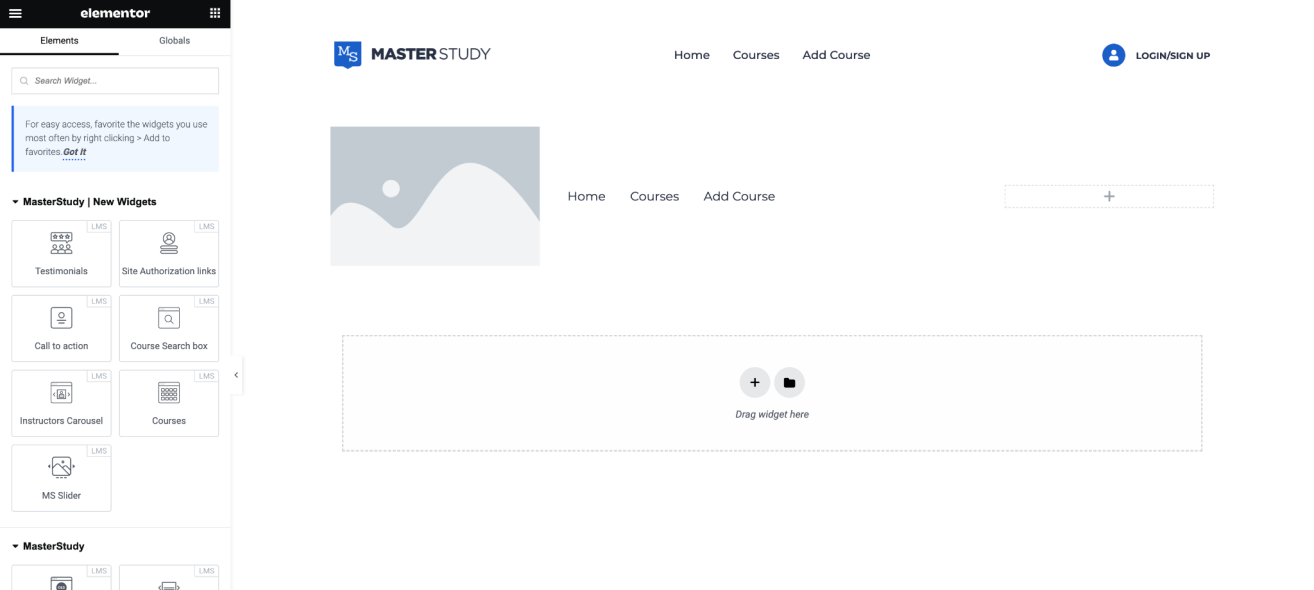The webpage for "Master Study" (MS) is laid out with multiple navigational and interactive elements. The top navigation bar features tabs labeled "Home," "Courses," and "Add Course." On the far right, there is a user profile photo icon accompanied by options to "Login" or "Signup." Below the navigation bar, there is a gray, dark gray, and light gray square, featuring a wave-like design.

The next row of tabs mirrors the first, including "Home," "Courses," and "Add Course," flanked by a rectangular box with a plus sign. Below this row is another interactive box with a plus sign within a circle and a folder icon within a circle, suggesting options to drag and add widgets.

To the left of these elements, there is a sidebar with a black-bordered hamburger icon labeled "Elementor." Below this, nine white square boxes are displayed, followed by tabs labeled "Elements" and "Globals." Further down is a search bar for user convenience.

The main section of the webpage is populated with various "Master Study" widgets, including a testimonial section, site authorization, course search box, call to action, instructions carousel, courses overview, and the MS slider. At the bottom, two additional widgets are noted, one resembling a printer. The webpage appears to serve as both a guide and a showcase of "Master Study" widgets and features.